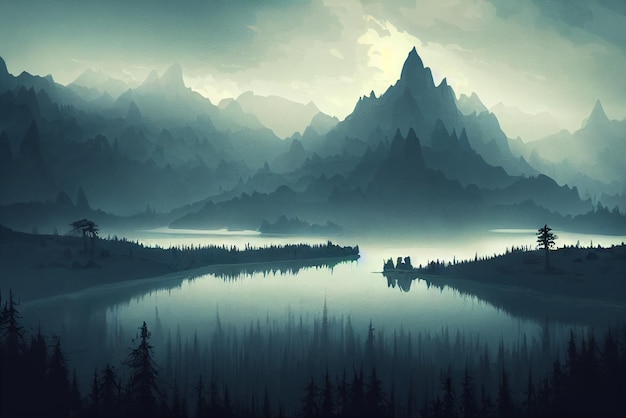This captivating outdoor image showcases a tranquil mountain and lake scene, portraying a daytime setting that could be a photograph, a painting, or a digital creation. The sky overhead is a misty blue, interspersed with white clouds, giving a slightly foggy ambiance. Dominating the background, a stunning mountain range features peaks with varying shades of blue, light blue, and off-white, creating a layered effect of overlapping mountain lines. In the foreground lies a serene lake, its surface reflecting the surrounding pine trees and jagged rocks that line its edge. The lake itself appears to split into two parts, converging and then diverging again. Along the shore and on pieces of land jutting into the water are clusters of pine trees and some smaller, younger trees. The serene water mirrors the intricate details of the landscape, completing this peaceful wilderness tableau.